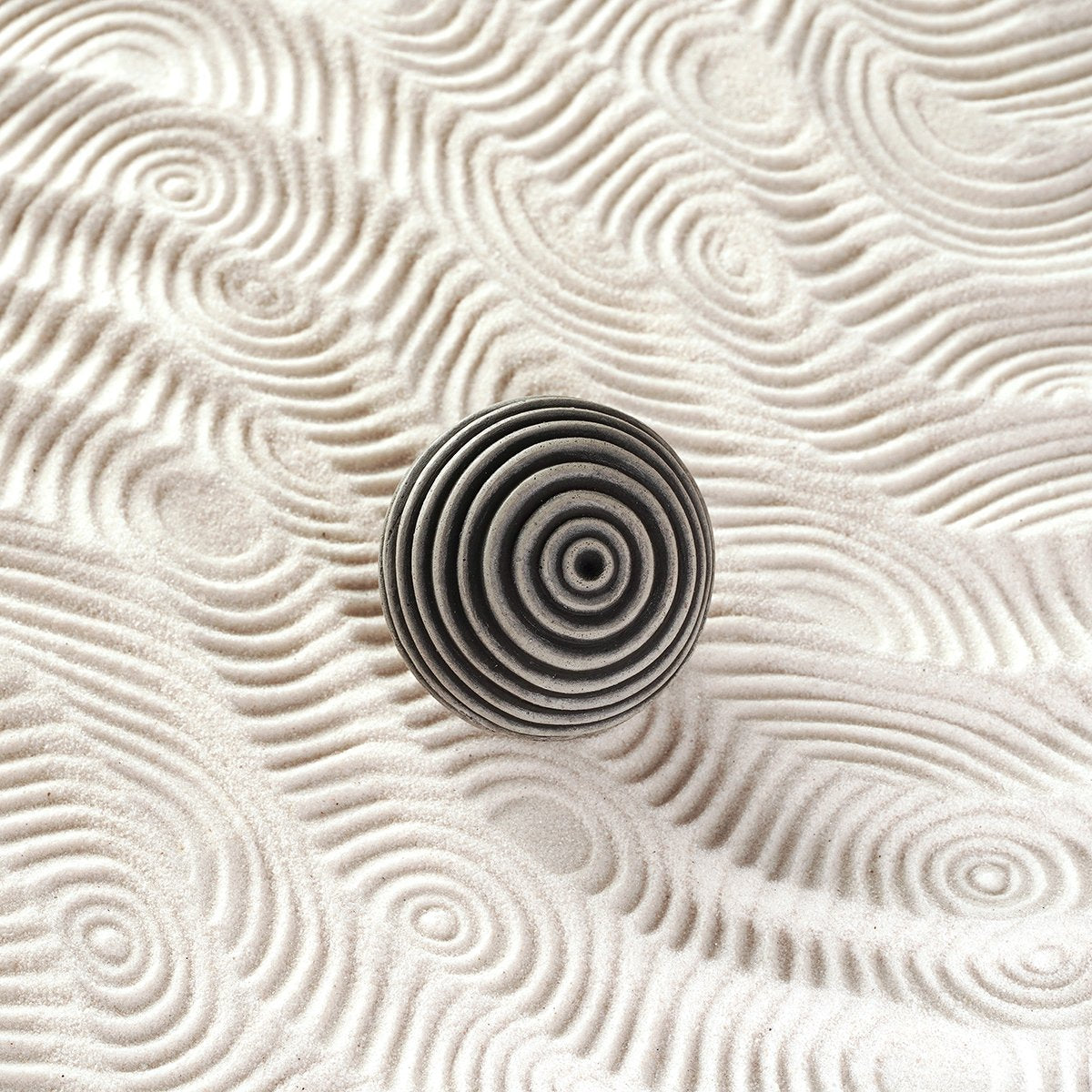In the image, there is a complex mosaic scene with a sophisticated background resembling a patterned mattress, adorned with intricate, curved, and swirly circular designs, akin to those crafted in sand. These patterns create a series of bumps and waves, contributing a sense of texture and depth to the backdrop. Nestled at the center of the image is a spherical object, which appears to be constructed from concentric circles that cascade and spiral outwards, enveloping the form of a ball. This ball is a dark slate gray color, with each ring slightly darker and casting subtle highlights along its edges. The sand-like background is a mix of light tans, whites, and darker shadows, enhancing the contrast of the dark gray ball. The circle and wave patterns etched into the sandy background add an intricate, decorative quality, as though drawn by hand with a tool, creating a harmonious blend of swirling patterns and repeating motifs.